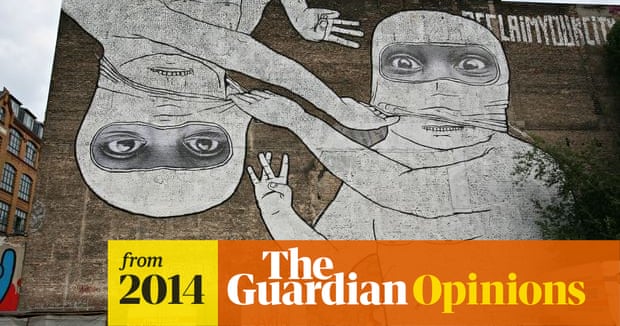The photograph captures a striking urban scene dominated by a brown, heavily textured brick building. The side of the building, devoid of windows or doors, is adorned with a large mural. The mural intriguingly depicts two cartoonish, humanoid figures, one hanging upside down and the other right side up. Both figures are dressed in white ski masks and appear to be unmasking each other. Uniquely, the masks' eyeholes reveal lifelike human eyes, as if from a photograph, adding a surreal touch to the artwork. The top right corner of the mural features the text "claim your city," while the bottom portion of the image is overlaid with a semi-transparent banner. This banner consists of a small yellow rectangle reading "from 2014" and an orange strip that states "The Guardian Opinions." The scene is set against an overcast gray sky, indicating the photograph is taken outdoors in a city. On the left, a glimpse of an adjacent orange brick building with numerous glass windows can be seen, adding context to the urban environment. Some graffiti is also visible at the bottom left of the mural, blending into the gritty cityscape.